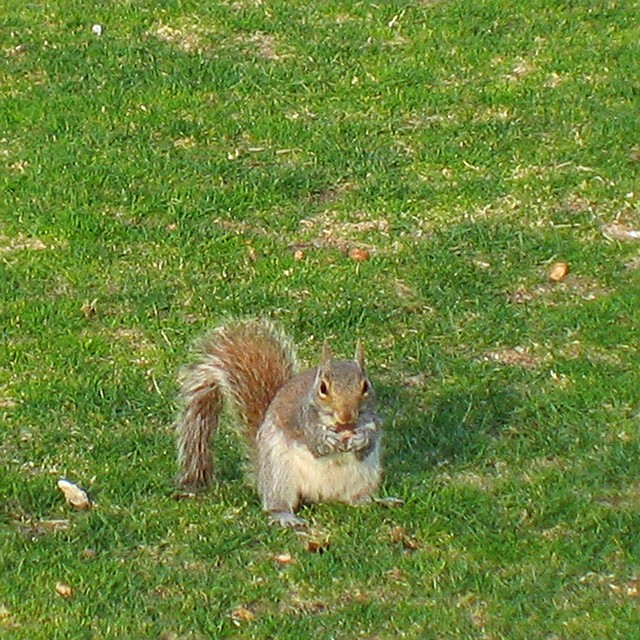A scenic outdoor photograph captures a chubby squirrel standing amidst lush green grass, munching on an acorn. The squirrel's position in the lower middle part of the image allows a clear view of its expressive face, with its black eyes keenly focused on the camera and ears perked up curiously. The squirrel's fur is a blend of brown and gray on its back and tail, while its belly showcases a lighter off-white or tan hue. The well-maintained grass dominates the scene, featuring several patches of brown, possibly from uneven growth, and a scattering of small leaves and sticks, adding to the natural charm of the setting.